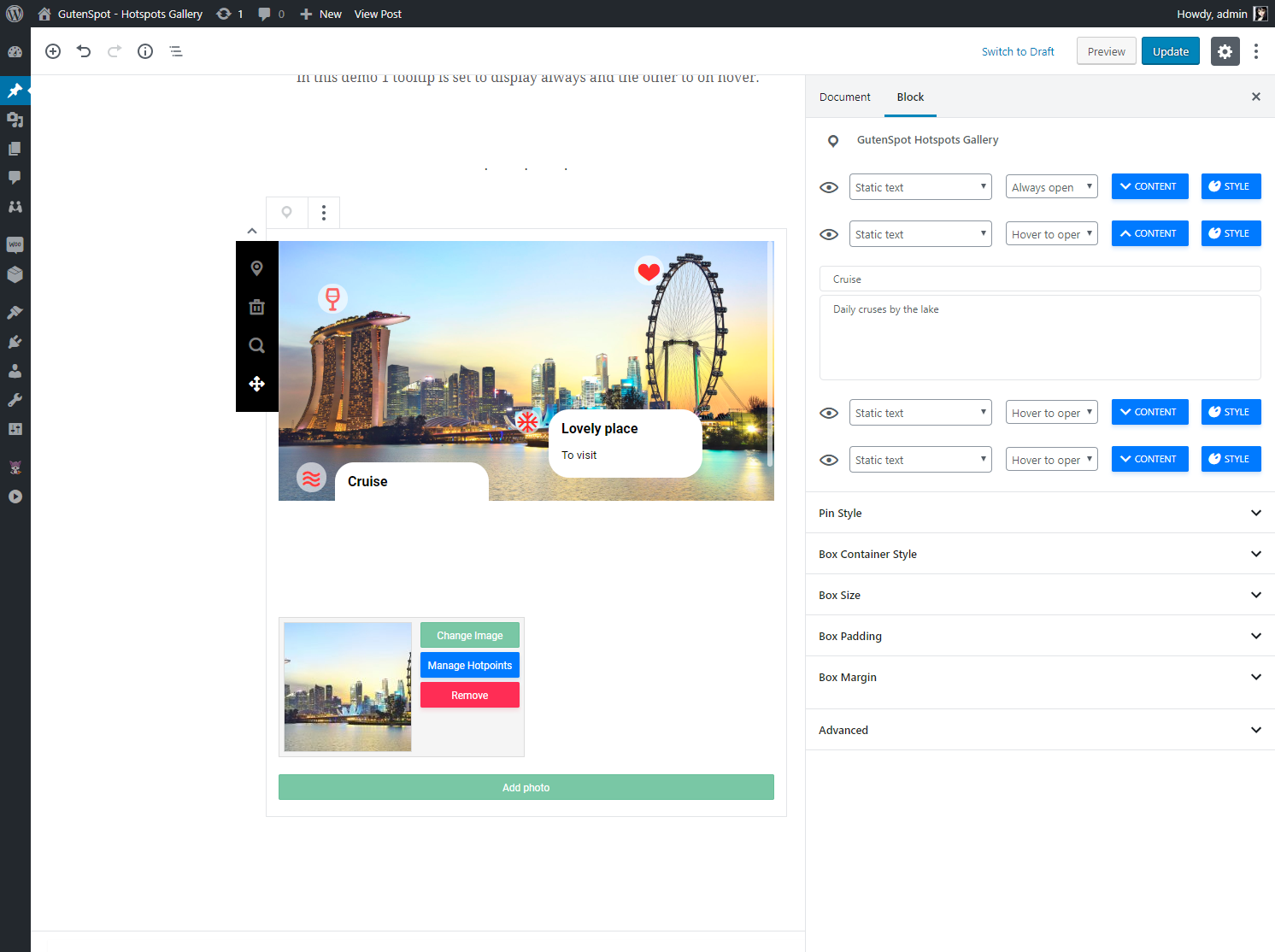The image depicts an open WordPress application, identified by the "W" logo on the top left. The interface is for a website builder. The right half of the screenshot showcases several controls, including toggle switches, dropdown menus, text fields, and tabs. These tabs include options for "Document" and "Block," while the interface options include buttons for "Draft," "Preview," "Update," and "Static Test." Additionally, there are various styling options such as "Pin Style Box," "Content Style Box," "Size Box," "Padding Box," "Margin," and "Advance" settings, located at the bottom right corner.

The left half of the image displays a visual preview of the website being constructed. The theme appears to be a scenic cityscape featuring a Ferris wheel against a backdrop of a blue and yellow sky, situated above a serene lake. There is a building on the left side of the image. At the bottom left, there is an interactive section with image management options, including icons labeled "Change Image," "Manage Hot Points," and "Remove." These options are color-coded with green, blue, and red backgrounds, respectively. Additionally, there is a green "Add Photo" button at the bottom of the image.